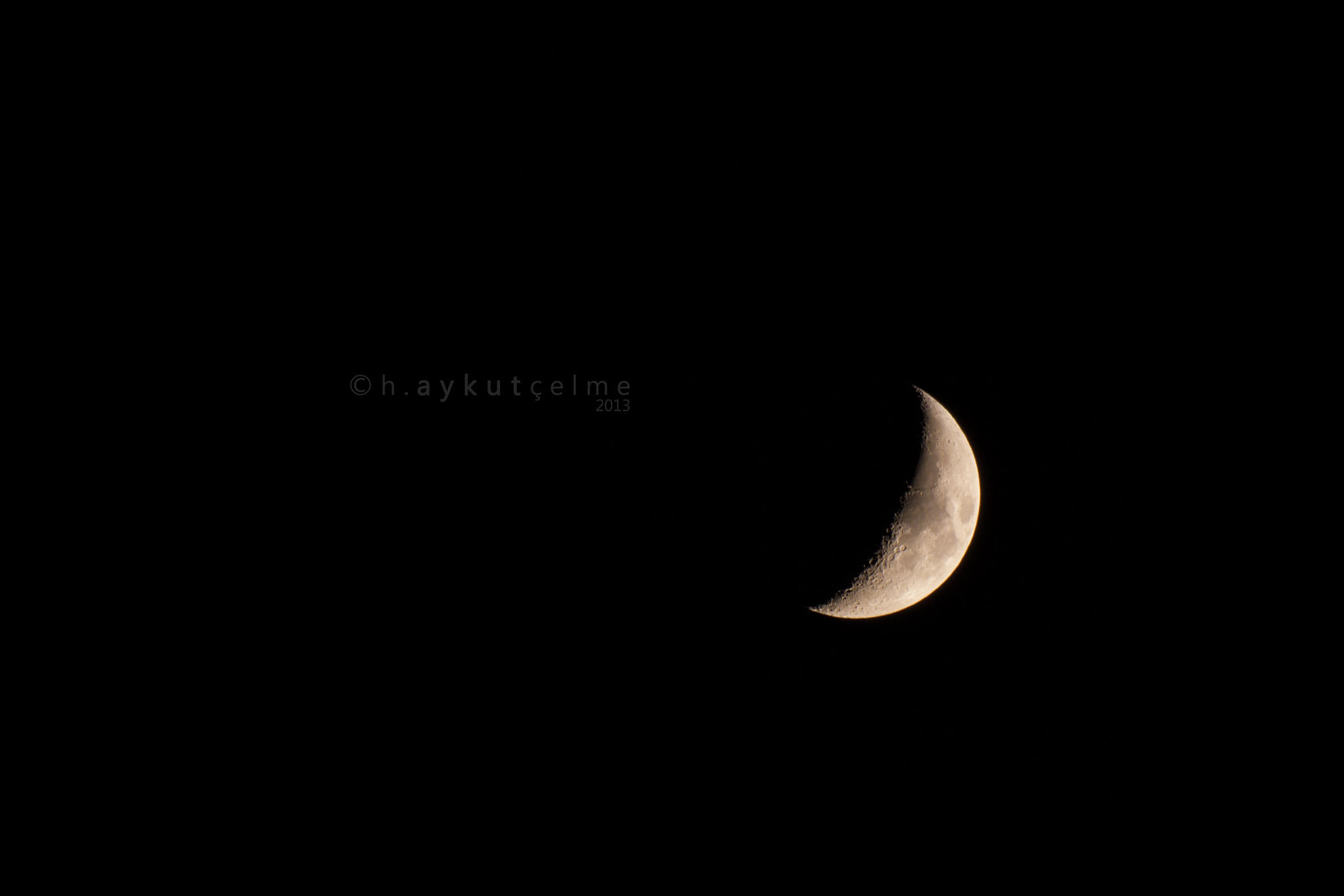The image depicts a pitch-black night sky devoid of stars, featuring a small crescent moon slightly left of center. The moon, in its crescent phase, reveals detailed gray and white craters across its pebbly surface. A subtle shadow accentuates its crescent shape. Superimposed on the dark backdrop, faint dark gray lettering is barely discernible, comprising a copyright symbol followed by "h.aykutcelme," with "2013" inscribed underneath in minuscule text.